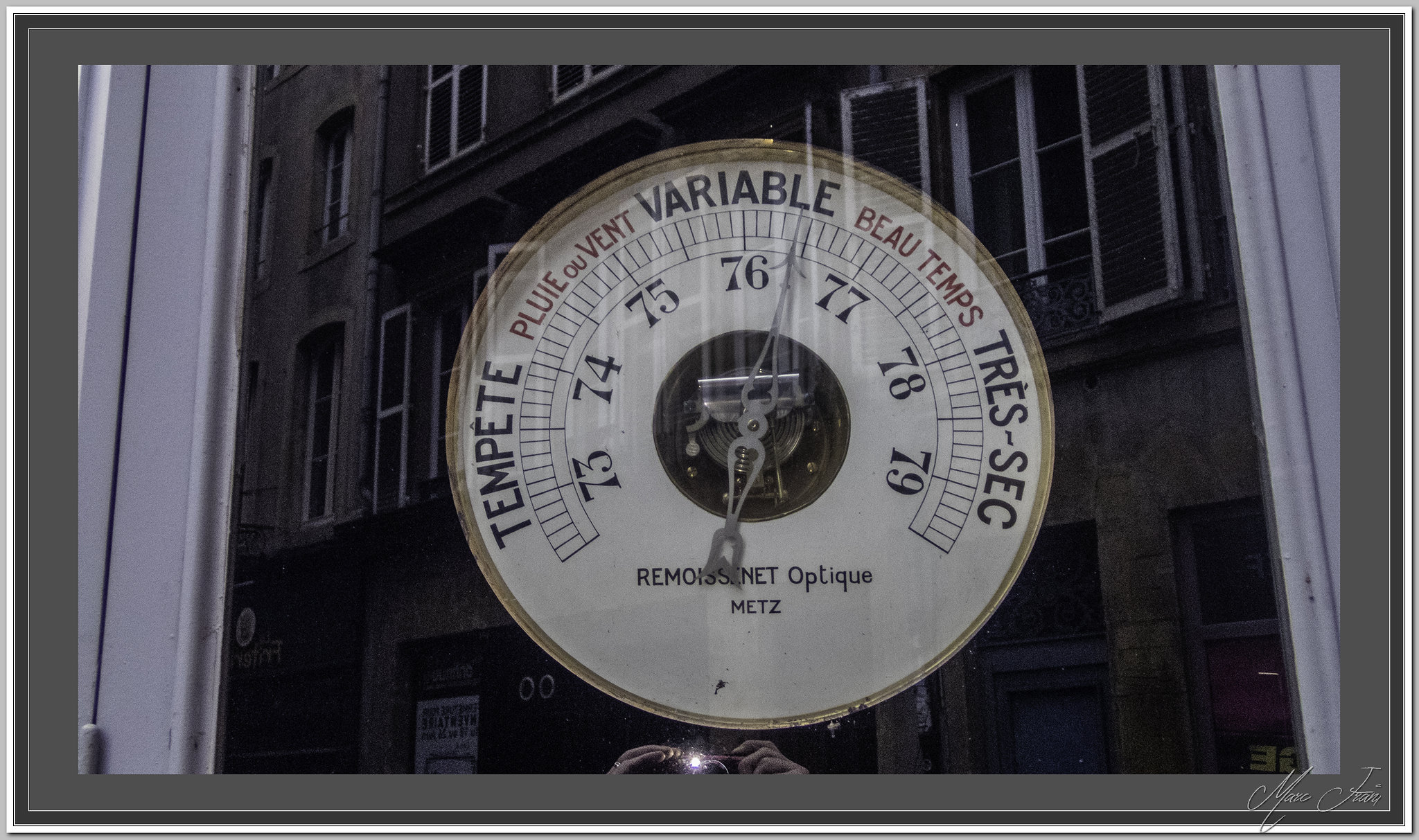The image depicts a temperature gauge branded as Metz, specifically designed for temperate regions. The thermometer, which appears to have a sleek white base with black text, has a large silver needle at its center. Notably, the gauge measures temperatures in the range of 73°F to 79°F, with ten individual interval marks between each degree for precise readings. The display features several terms such as "Temptique," "Pouvent" (highlighted in red), "Variable," "Beaux-Temps" (also in red), "Très Saint," and "Reminiscent Optique." These terms emphasize various weather conditions and temperature sensations, providing a comprehensive reference for users. The overall design is both functional and aesthetically tailored for moderate climates.